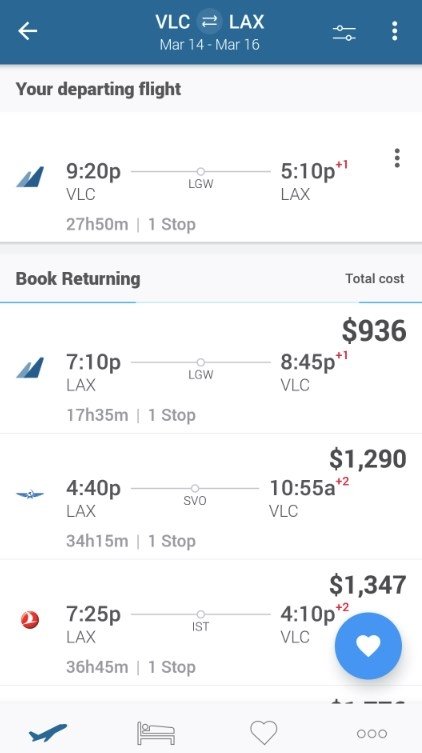Screenshot of a Flight Schedule:

The image is a screenshot of a mobile phone display, depicting an individual's flight schedule in a long rectangular format. At the top of the screenshot, there is a dark blue header featuring an arrow pointing to the left labeled "VLC," flanked by two arrows pointing in both directions labeled "LAX," and the dates "March 14th - March 16th." On the right side of this header, there are icons for a sort/filter option and a vertical ellipsis (three dots) for additional options.

Below the header, the schedule details begin with a segment indicating the departing flight from VLC at 9:20 p.m., stopping at LGW, before continuing to LAX, arriving at 5:10 p.m. the next day (+1 day). This leg of the journey totals 27 hours and 50 minutes with one stop.

Further down, under the section labeled "Book Returning," several return flight options are listed:

1. 7:10 p.m. departure from LAX, arriving at VLC at 8:45 p.m. the next day, totaling 17 hours and 35 minutes with one stop, priced at $936.
2. 4:40 p.m. departure from LAX, arriving at VLC at 10:55 a.m. the day after next, totaling 34 hours and 15 minutes with one stop, priced at $1,290.
3. 7:25 p.m. departure from LAX, arriving at VLC at 4:10 p.m. the day after next, totaling 36 hours and 45 minutes with one stop, priced at $1,347.

At the bottom of the screenshot, there are icons for a heart inside a circle (indicating favorite/like), a plane symbol, a hotel icon, and another vertical ellipsis (three dots) for more information.